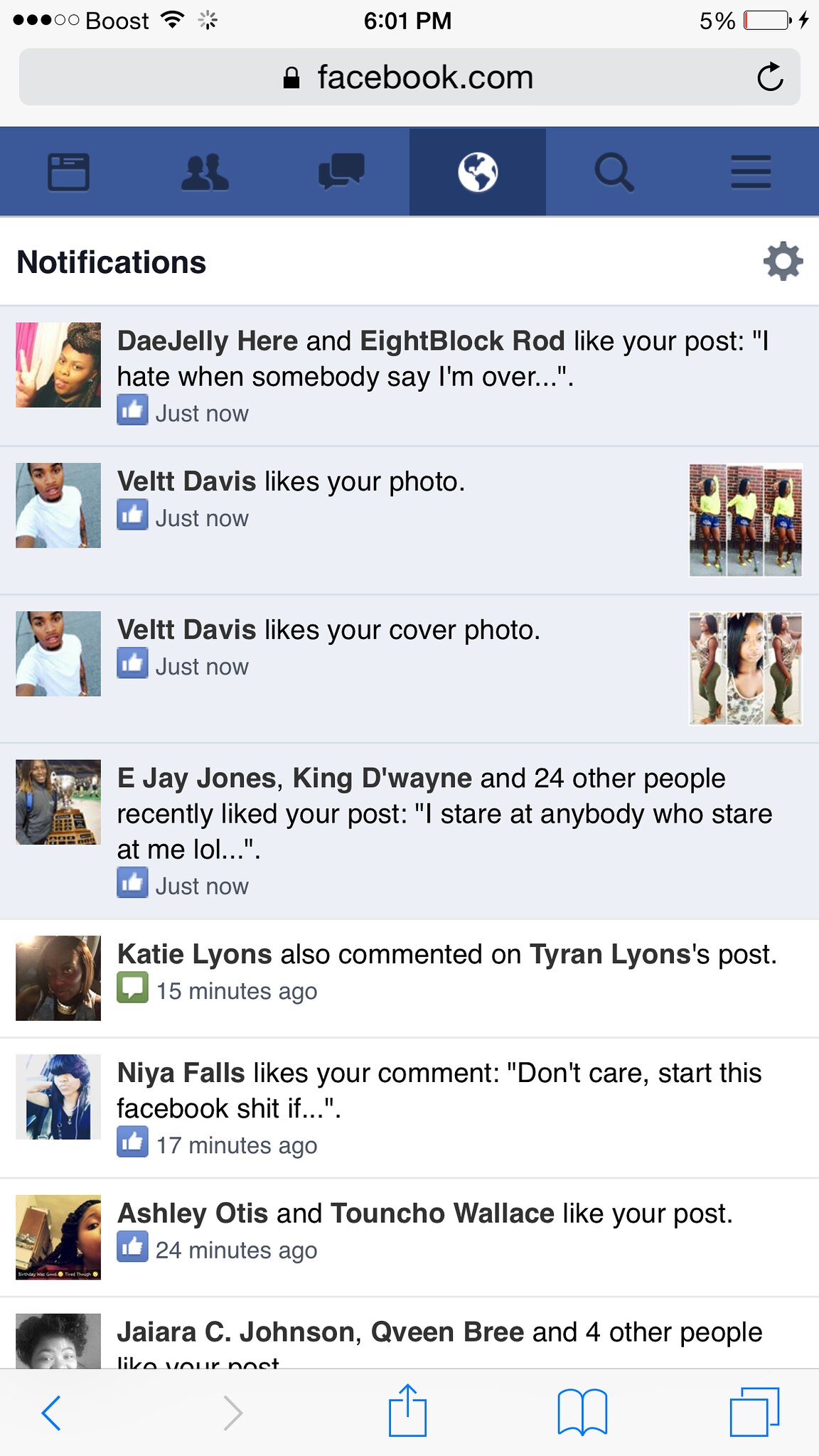The image is a detailed screenshot of a Facebook notification screen on a smartphone. At the top of the screen, the status bar shows the "Boost" network with full signal, the time "6:01 PM" prominently in the center, and a nearly depleted battery at 5% on the top right corner. Below the status bar is the URL bar indicating the secured site, "facebook.com," followed by a navigation bar with various Facebook tab icons like Photos, People, Comments, World, Search, and a dropdown menu. 

Underneath, the notifications section displays several interactions:
1. Dave Jelly and 8th Block Rod like a post that says, "I hate when somebody says I'm over."
2. Vilt Davis likes a photo and also likes a cover photo, each shown with corresponding images.
3. E.J. Jones, King Duane, and 24 others liked another post stating, "I stare at anybody who stare at me, LOL."
4. Katie Lyons commented on Tyren Lyons' post 15 minutes ago.
5. Nia Falls liked a comment that reads, "Don't care, start this Facebook shit if…," 17 minutes ago.
6. Ashley Otis and Townshow Wallace liked a different post 24 minutes ago.
7. Jayara C. Johnson and four others liked another post, though the message is cut off by the bottom navigation bar.

The bottom navigation bar consists of a back arrow highlighted in blue, a forward arrow in gray, a share icon, a library icon, and an icon depicting two overlapping squares, typically indicating open tabs.